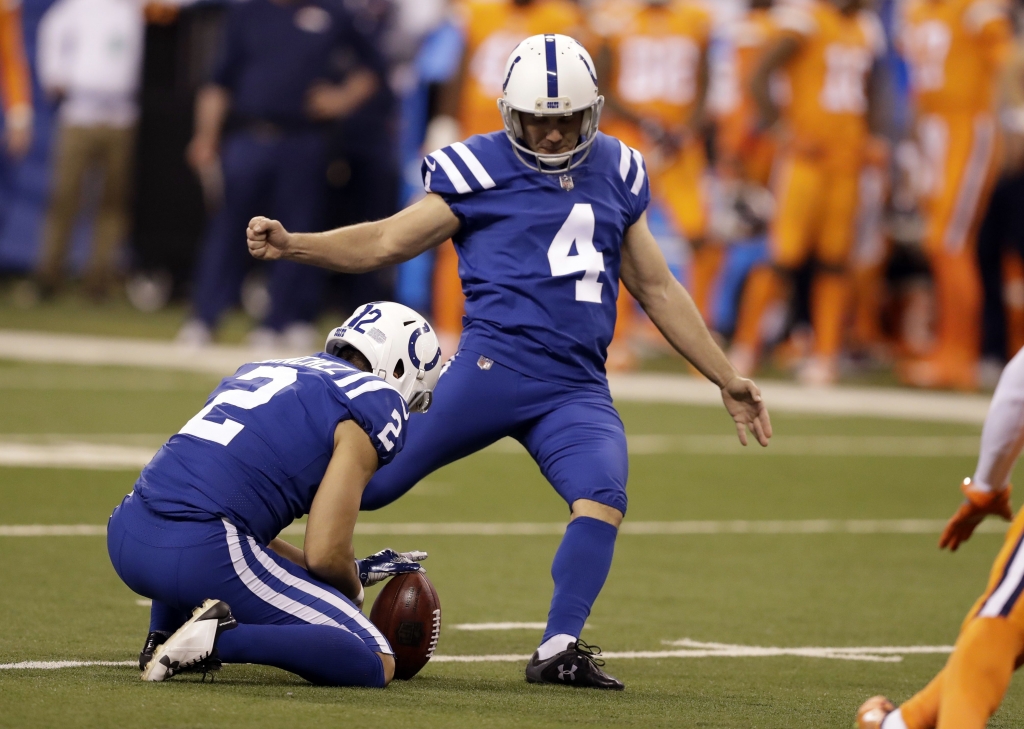The rectangular, horizontal image captures a pivotal moment during an American football game, specifically during a kickoff. Central to the scene are two players from the Indianapolis Colts, distinguished by their blue jerseys featuring white stripes on the shoulders and sides, and white helmets adorned with the Colts' iconic horseshoe logo. The kicker, wearing jersey number 4 and sporting black shoes, is in mid-kick, his right leg poised and ready to strike the football. To his left, the holder, donning number 12 on his helmet and wearing white shoes with black accents, is steadfast on the ground, ensuring the football is perfectly positioned for the kick. In the background, a group of players in orange uniforms—and some in casual clothing—watch intently. Additionally, the legs of an opposing player in orange gear with black and white stripes are visible in the bottom right corner, potentially indicating an attempt to block the kick.